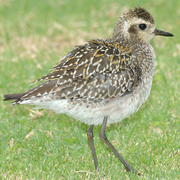This outdoor photograph features a young Pacific golden plover standing upright in a grassy field. The bird, centrally positioned, has a plump, round body with thin, bent-down legs, although its feet are obscured by the grass. Its back feathers are predominantly dark brown, speckled with beige and yellow spots, while its underside is white. It has a light brown neck and a head adorned with a mix of dark brown and beige, with dark brown around its black, beady eyes that glance to the right. Its thin, long black beak is also directed to the right. Despite the low resolution and blur, it's clear the bird's surroundings fade into a blurry backdrop, emphasizing its solitary presence in the image.